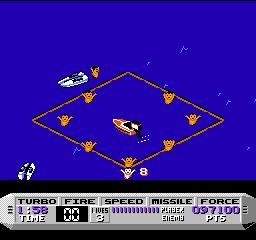This image is a screenshot from a video game primarily featuring a royal blue body of water. At the center of this water scene is an orange diamond shape with several floating orange items that resemble creatures with their arms extended upward. Inside the diamond, an orange and white motorboat is prominently displayed. Outside of the diamond and towards the upper left corner of the frame is a white boat, while another white boat is positioned in the bottom left corner. 

At the bottom center of the diamond, a white creature mirroring the orange ones with arms extended is noticeable. To the right of this creature, the number "8" is displayed in white. The bottom portion of the image contains the game's score information. The words "Turbo," "Fire," "Speed," "Missile," and "Force" appear in black font against a gray background.

Below these labels, the screen shows a time of "158," with "00 lives," followed by the digits "3," "0," "9," "7," "100 points." The text "Premier Games" is displayed in purple and white font against a gray background, all framed by a black border.